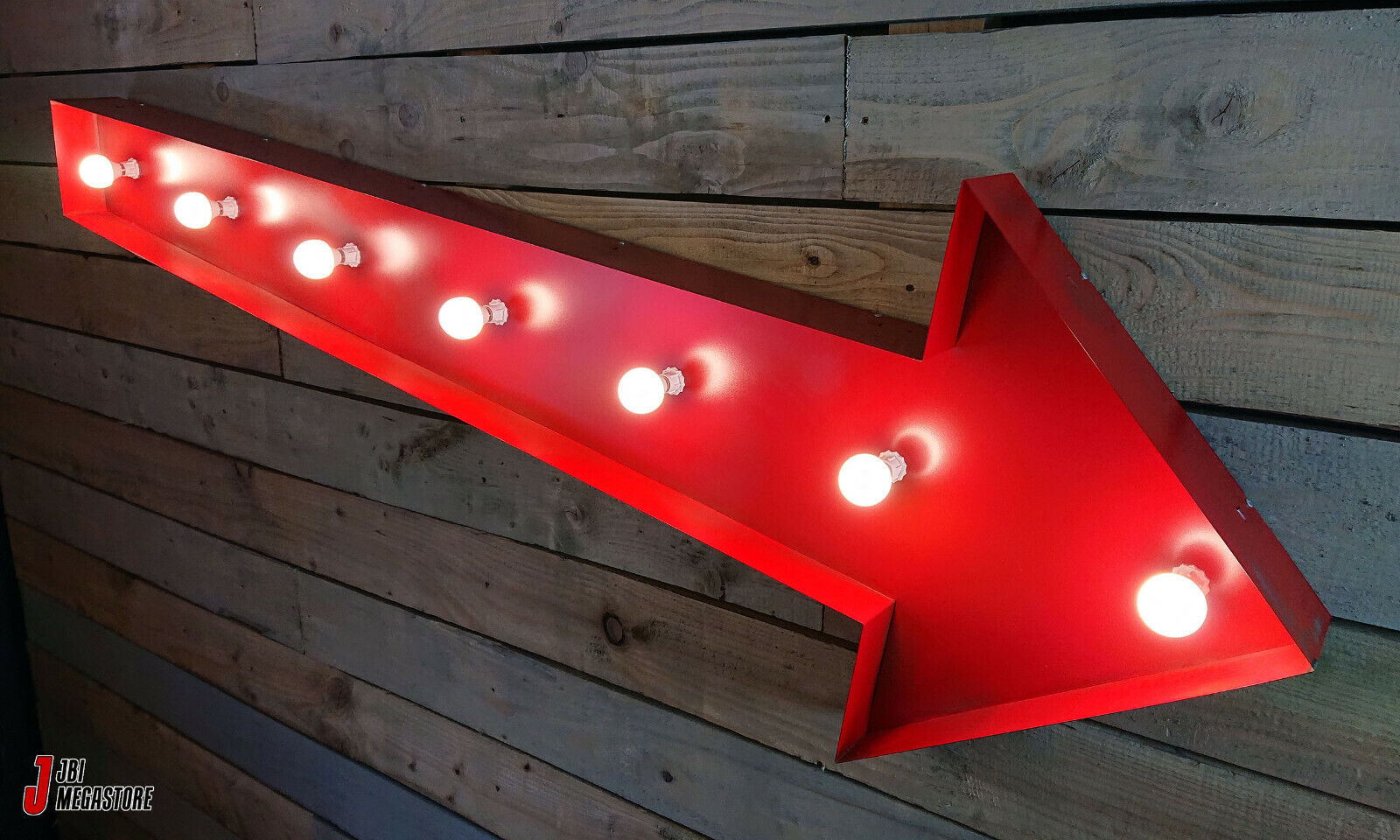This photograph showcases a striking Art Deco style, long red metal arrow mounted on an unfinished wooden wall with visible plank gaps, resembling a barn aesthetic. The arrow, pointing from left to right, serves as a frame for seven illuminated light bulbs embedded in its indented center, each casting a half-circle reflection on the arrow. The photograph captures the arrow angled such that its tip is near the bottom right corner, highlighting the contrast between the arrow's vibrant red hue and its dark black top. A logo featuring a red "J" and the text "JBI Megastore" in black with a white outline is visible in the left foreground, adding a subtle commercial element to the image.